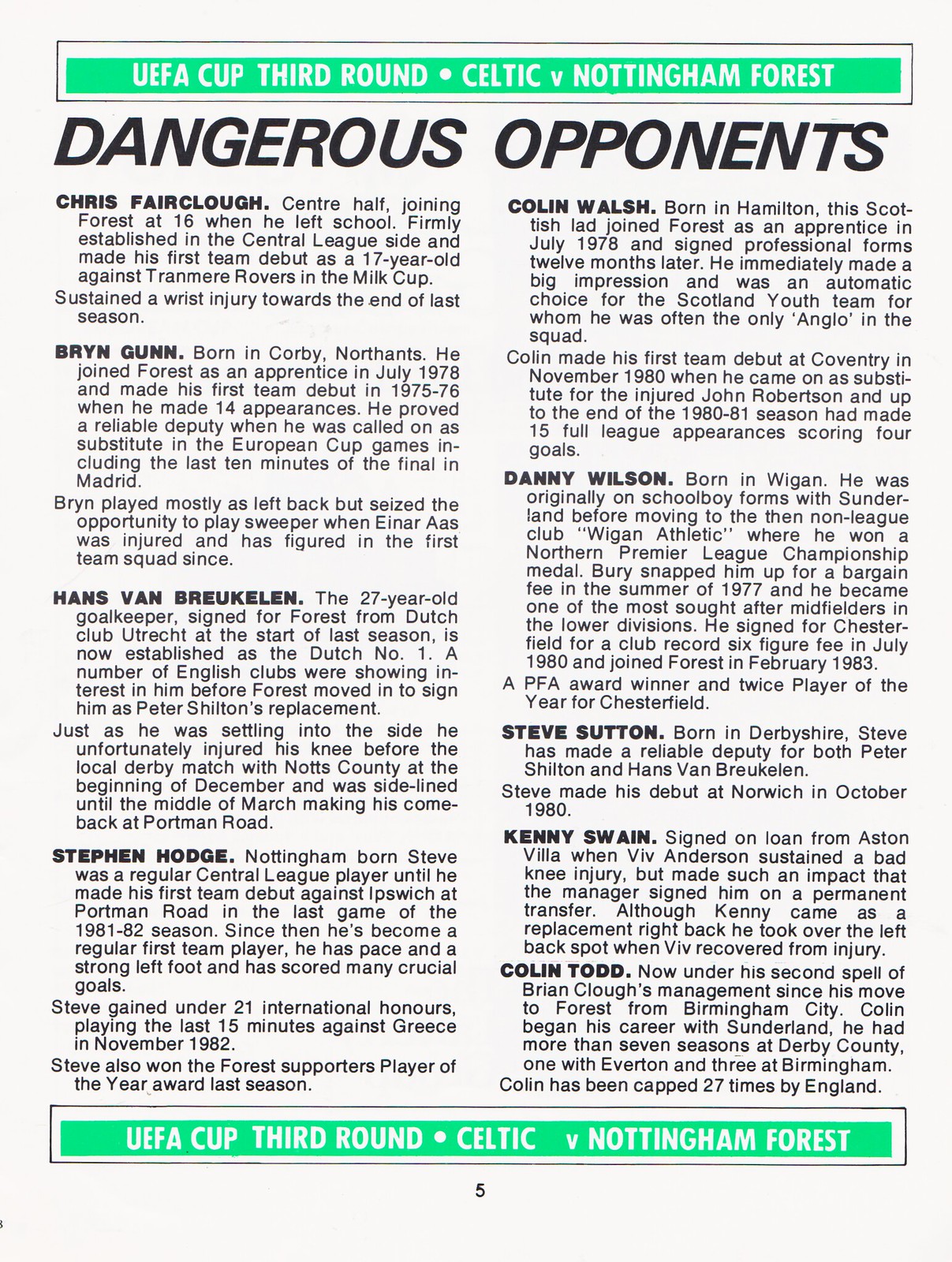The image, appearing as a page from a sports magazine, is set against a light green backdrop with a rectangular portrait orientation. At the top, a green horizontal strip features the text "UEFA Cup 3rd Round Celtic vs. Nottingham Forest" in white letters, which is repeated again in the footer strip at the bottom of the image. Centrally positioned at the bottom is the number 5.

Prominently displayed below the top strip, in bold black capital letters, is the heading: "Dangerous Opponents." The main body of the page contains several paragraphs of detailed text, formatted into two vertical columns. Key names and phrases are in bold black print, including players such as Chris Fairclough, who joined Forest at 16 and made his first team debut as a 17-year-old, Bryn Gunn, Hans van Breckelen, Stephen Hodge, Colin Walsh, Danny Wilson, Steve Sutton, Kenny Swain, and Colin Todd. This richly detailed page encapsulates a comprehensive analysis of the teams and their players, fitting snugly into the visual aesthetic of a sports magazine.